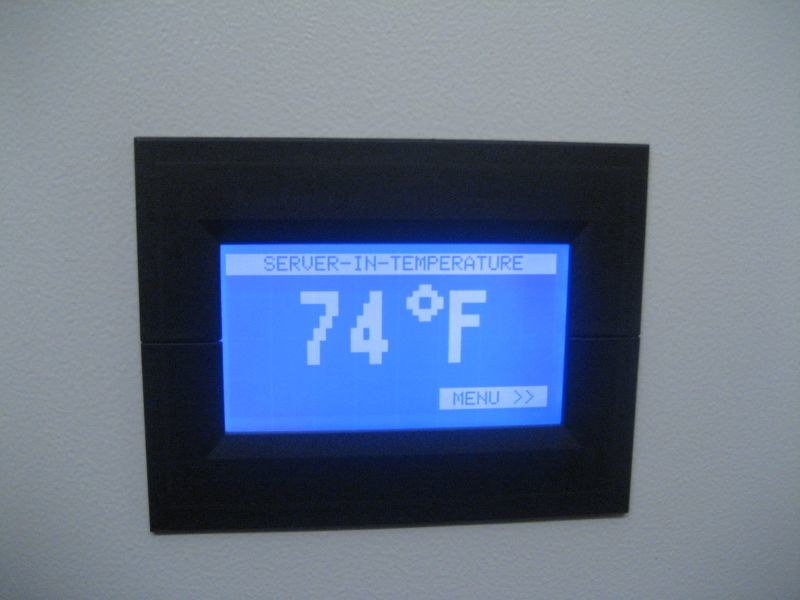The photograph showcases a digital temperature display mounted on a white wall. The display is encased in a thick black frame, which is of a basic and low-resolution design. The screen features a blue background with a white bar at the top, containing blue text that reads "Server-In-Temperature". Below this, large numbers "74" are prominently displayed, followed by a degree symbol and the letter "F" for Fahrenheit, indicating the temperature. In the bottom right corner, there is a smaller white bar with blue text that says "Menu" along with two right-pointing arrows.